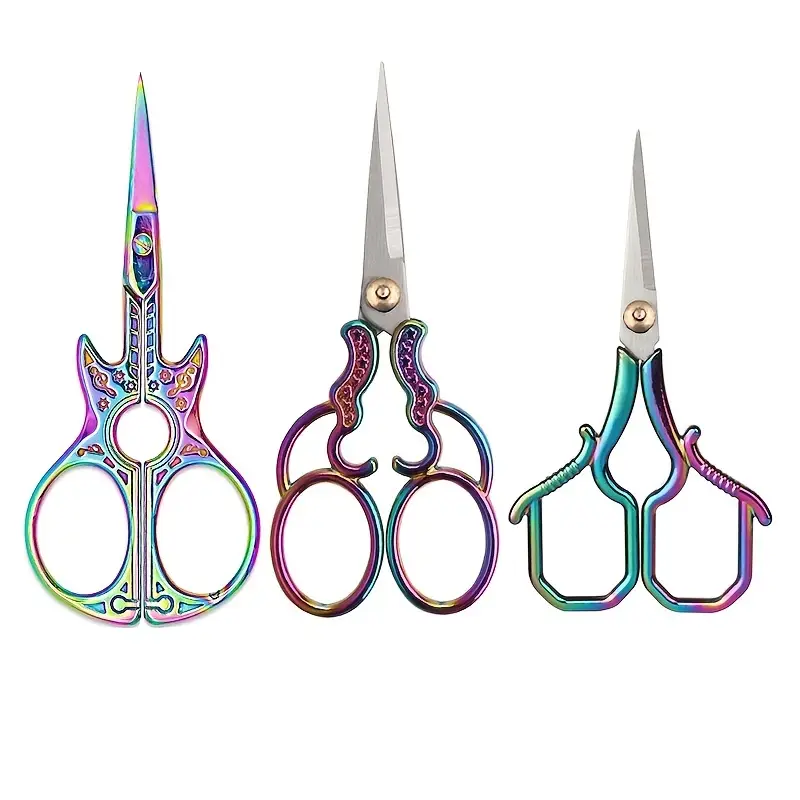This image presents three pairs of artistic and ornate scissors arranged vertically with their points facing upwards, set against a white backdrop. Each pair displays a unique and intricate design with iridescent handles that blend shades of blue, purple, green, and teal in a lustrous, ombre finish.

The pair on the far left is shaped like a guitar, featuring a pink handle with blue and yellow highlights, complete with a sound hole cutout and two large circular holes forming the guitar body for finger placement. The blades are sharp and seamless from top to bottom.

The middle pair of scissors has silver blades attached to beautifully curved handles, adorned with a vibrant mix of red, blue, and green. The handles are long ovals connected to the blades with thicker, squiggly lines that add an artistic touch to the whole piece.

The pair on the far right showcases a more angular design with silver blades and handles in fluorescent teal, purple, and green hues. The handles feature a unique square-circle shape with notches for grip, and above the finger holes, there's a melted screw-like detail that adds to its quirky charm.

Overall, these scissors combine functionality with a striking design, making each pair a piece of art in itself.